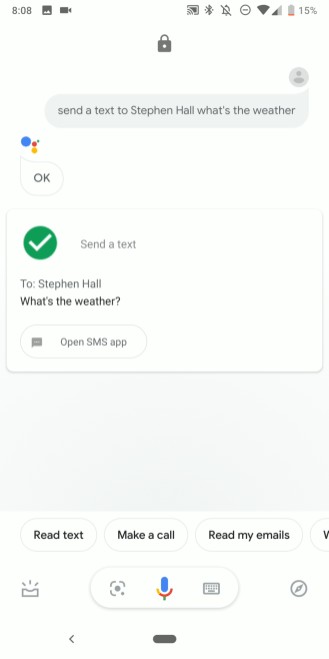This is a detailed screenshot of a smartphone interface. 

In the top left corner, the time reads "8:08 AM," with a slightly blurry and small video camera icon next to it. The top right corner features various status icons: Bluetooth, a crossed-out notifications icon, a circled icon with dots, a wireless connection symbol, a cellular signal icon, and a battery icon displaying a red sliver, indicating 15% battery life.

Centered on the page is a prominent black padlock image. On the far right, there is a gray circle containing a darker gray silhouette of a person. Beneath this, in gray text, it reads, "Send a text to Stephen Hall. What's the weather?"

Below this section are four circles: a larger blue circle, a significantly smaller blue circle, a red circle, and a yellow circle. Within a speech bubble, the text "Okay" is displayed.

Further down, there is a rectangular box featuring a green circle with a white checkmark. Accompanying this, it says, "Send a text to Stephen Hall," followed in bold by the command "What's the weather." Underneath, it reads, "Open SMS app."

At the bottom of the page, three horizontal options are displayed: "Read text," "Make a call," and "Read my emails." Below these options are a few icons, including a blue microphone and a keyboard icon.